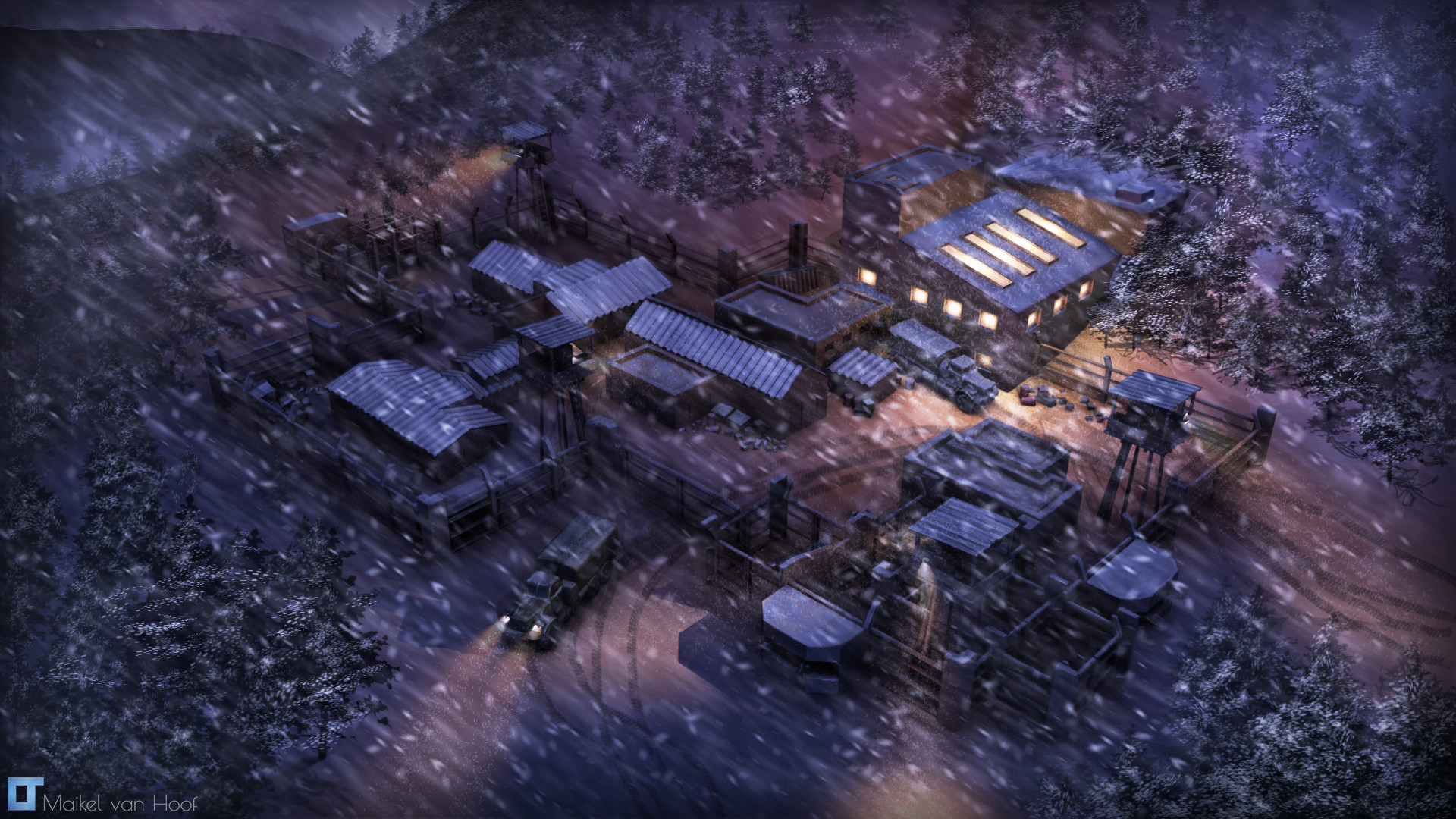This illustration, possibly a digital artwork or a screenshot from a video game, presents a bird's-eye view of a snow-covered town at night. The snowy scene features numerous buildings, mainly rectangular and one distinctly L-shaped, with some having skylights on their roofs. The largest structure, a gray warehouse with glowing yellow windows, is situated towards the top right corner, indicating activity inside. Snowfall is depicted as delicate, scattered dots across the scene, adding to the tranquil yet cold atmosphere of the night. Amidst the dark hues of black, dark gray, and purple, two sources of light stand out: the warehouse windows and the headlights of a large truck driving out of a fenced compound, leaving visible tracks in the snow. Located in the front and center of the image, the compounds are surrounded by a fence, with trees lining the perimeter, enhancing the sense of isolation and depth. The artwork is signed "M-A-I-K-E-L Van Hoof" at the bottom left.